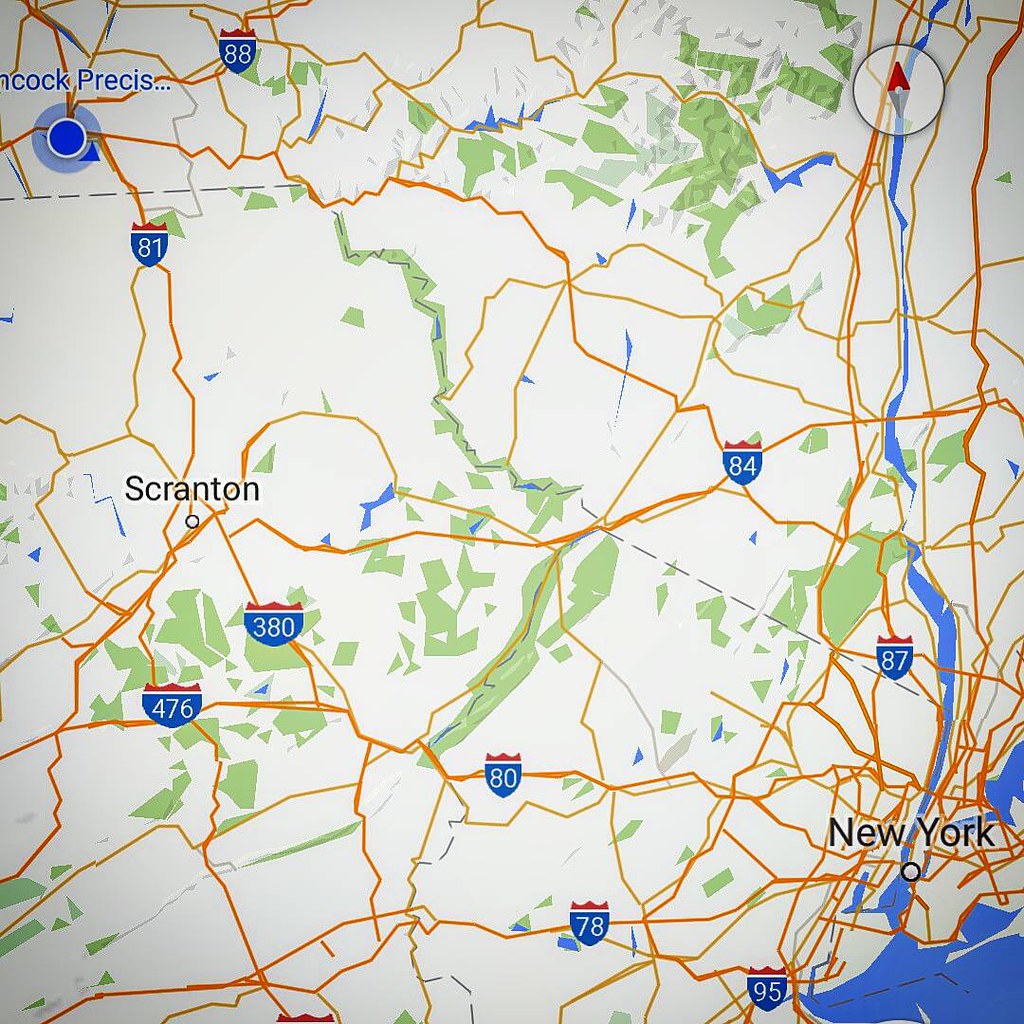The image features an online map primarily depicting the Scranton, Ohio area, extending to the right with New York City visible. The map has a predominantly light beige or off-white background interspersed with green areas representing parks or forests, and blue regions indicating rivers, streams, and lakes. Notable cities like Scranton and New York are highlighted. Various interstate highways, specifically 81, 380, 476, 84, 78, 95, 88, and 87, are marked with their distinctive blue and red shield icons with white numbers. Traffic conditions are indicated with red lines for heavy traffic and yellow for lighter traffic. Additionally, in the top left corner, a destination labeled “Hancock Precision” is marked in blue, while the upper right corner features a compass with a red arrow pointing due north.